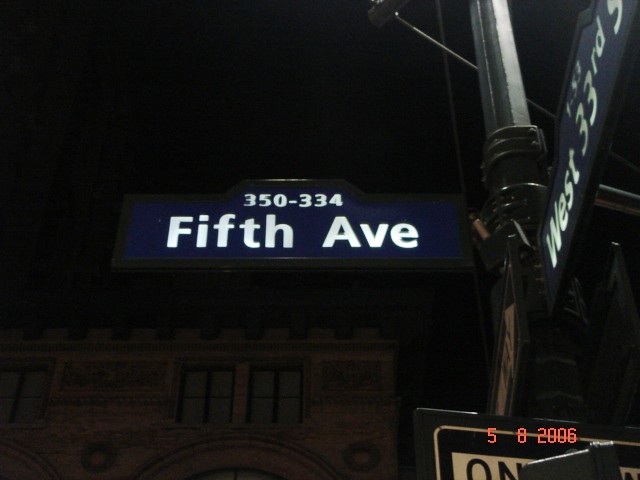A landscape-oriented photograph captures a street junction, likely in New York City, evidenced by the timestamp on the image of May 8, 2006. The perspective is upward, focusing on intersecting street signs. Prominently, the sign in the foreground states "350-334 5th Avenue." To the right, slightly behind the photographer's position, another sign indicates "West 33rd Street," its number partially obscured. Below these, a one-way street sign points to the right. This intersection is situated near the iconic Empire State Building.